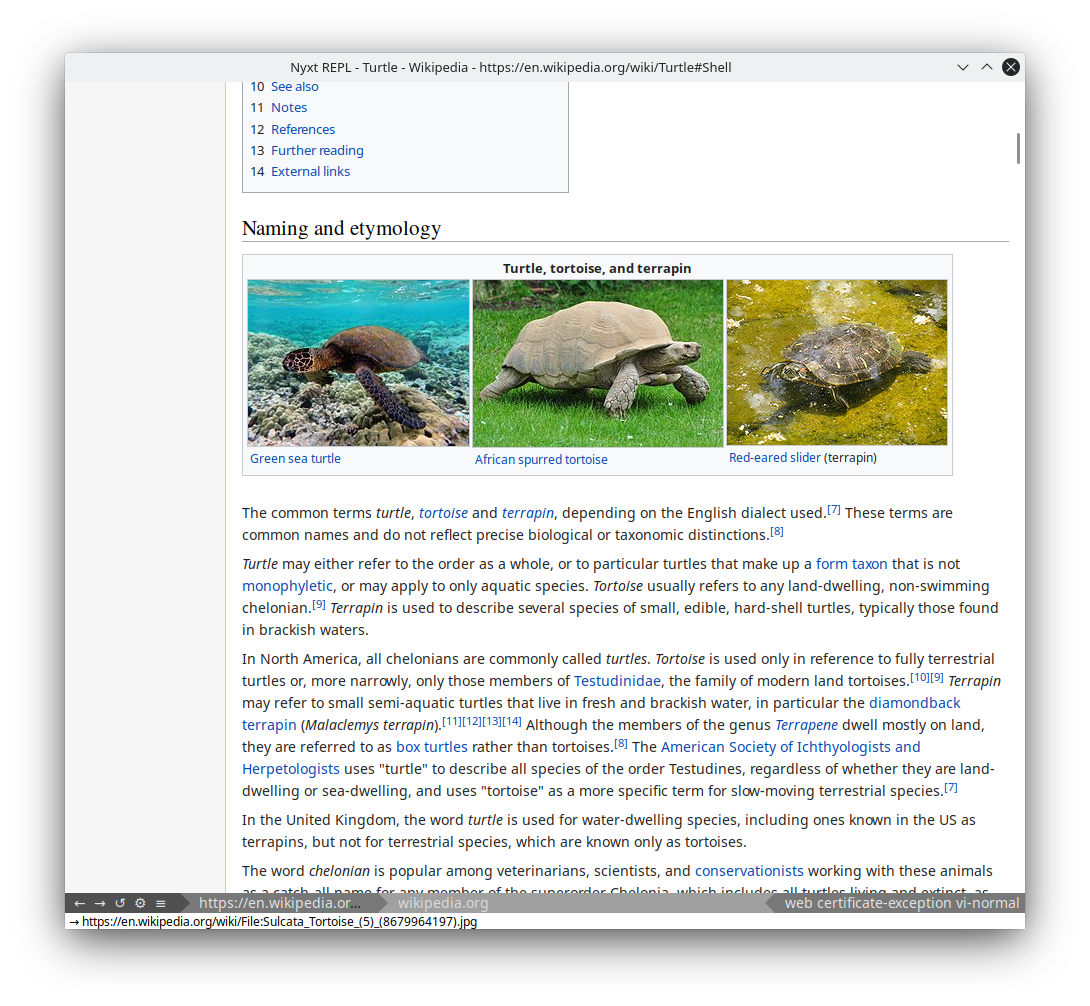The image is a screenshot of a Wikipedia page dedicated to the etymology of turtles. Dominating the foreground are three clear images of turtle species, specifically a turtle, a tortoise, and a pterygian, each showcased from different angles. The turtle on the left is angled towards the right, the tortoise on the right is angled towards the left, and the pterygian in the middle is facing forward. 

The background adheres to the standard aesthetic of Wikipedia, featuring a clean white canvas with black text and various blue hyperlinks. These hyperlinks direct readers to additional Wikipedia pages for more in-depth exploration of related topics. The page is structured with sections that include notes, references, further reading, and external links, providing exhaustive details on the etymology of turtles.

Furthermore, the text comprehensively covers common names and descriptions of turtles, detailing how to refer to various species. The primary focus is on North American research, with some references to studies conducted in the United Kingdom. The article delves into the history and linguistic roots of terms used to name and describe turtles and their species.